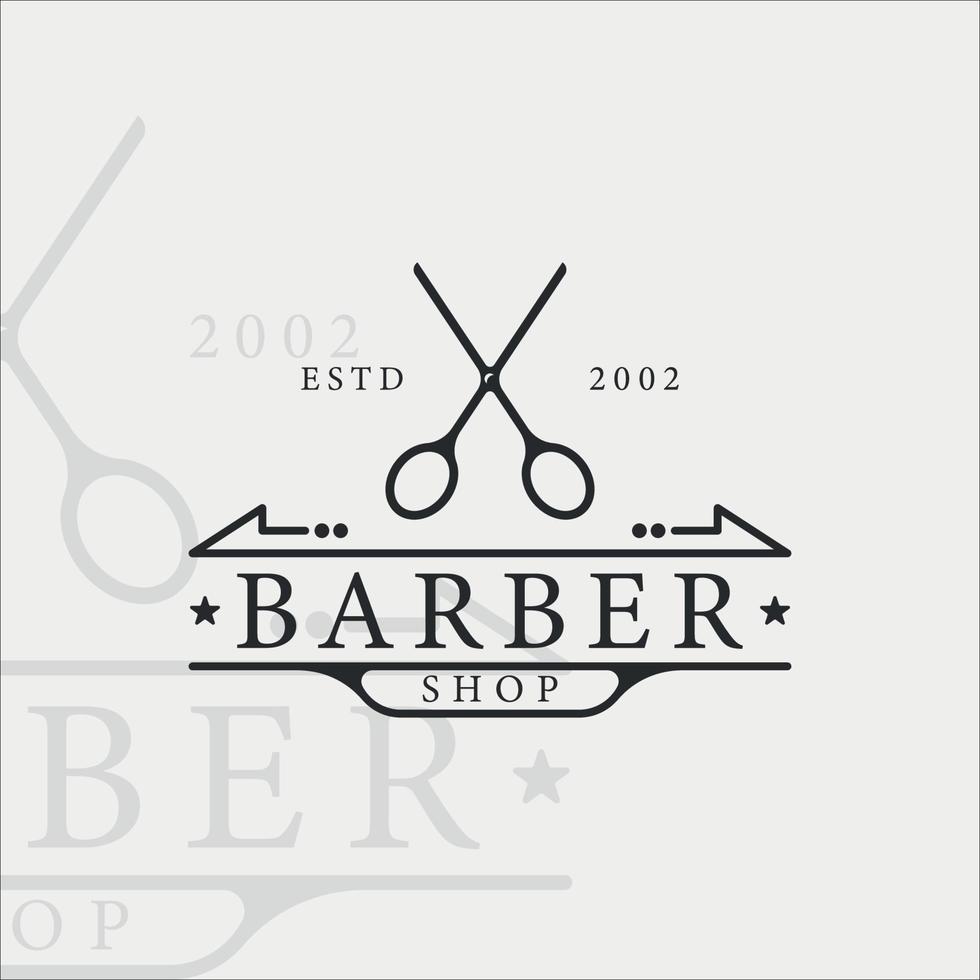The image depicts a detailed and artistic barbershop logo. At the center, a prominent pair of black scissors is featured, surrounded by stylized text. The word "ESTD" is written in all capital letters at the top, followed by "2002," indicating the establishment year. Directly below the scissors, "Barbershop" is displayed in black, flanked by two stars on either side, one near the “B” and the other near the “R” in "Barbershop".

Additionally, the logo incorporates a lighter gray overlay, slightly offset to the left, repeating the main elements including "BER" and "OP" with "2002" positioned at the bottom left. The entire design is set against a white background, with dark blue accents and elements of calligraphic styling. The overall composition is enhanced with graphic arrows and lines pointing to the left and right, adding a dynamic feel to the advertisement.